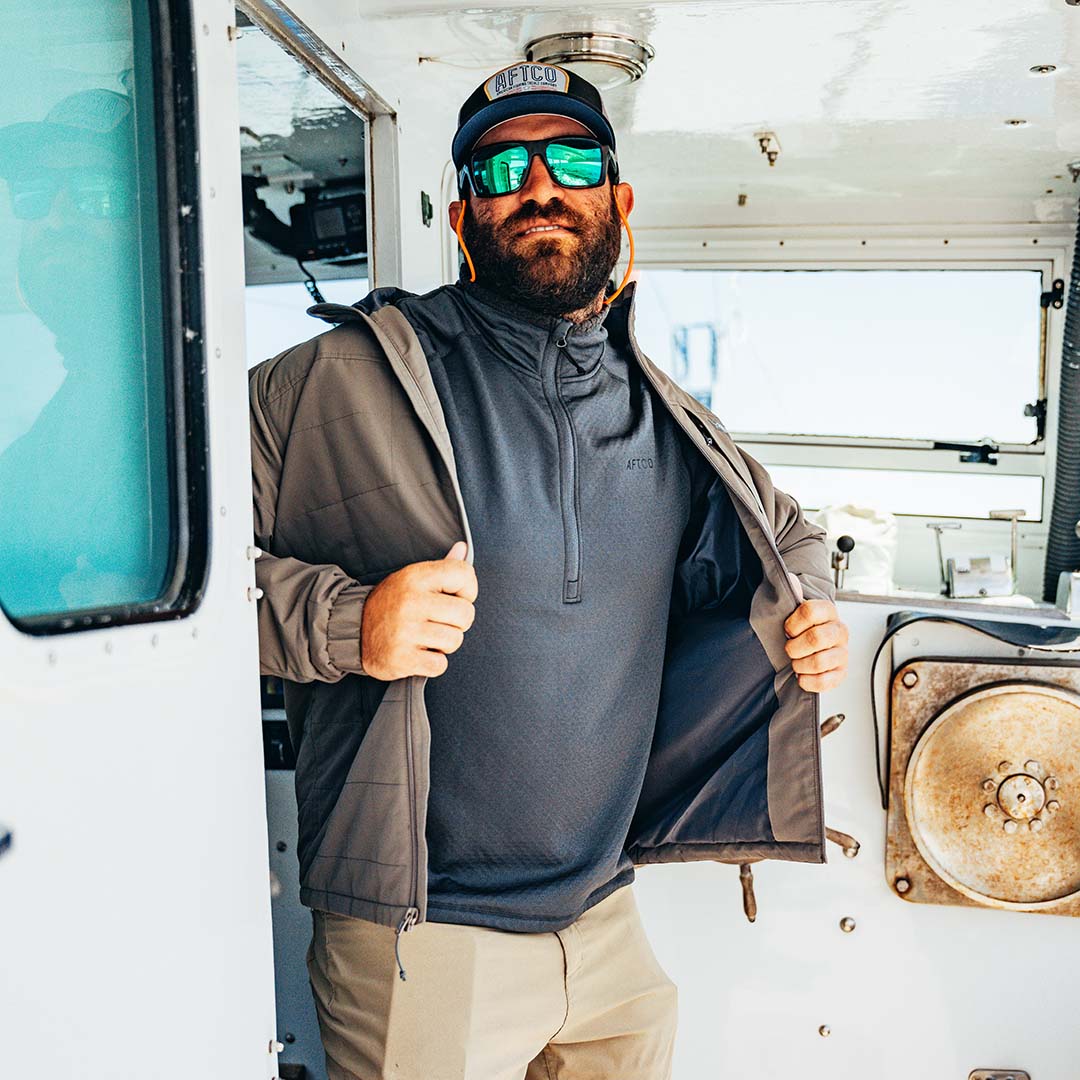In the image, a man stands in the cab part of a boat, suggesting an interior setting with a nautical atmosphere confirmed by visible communications equipment behind him. He appears to be the captain, positioned near the wheel and gazing at the camera with a half smile. Sporting a thick, full beard and mustache, he wears a black baseball cap with a blue underside and a white patch bearing the letters "AFTCO." His eyes are shielded by reflective blue sunglasses with black rims, secured by an orange sunglass holder around his neck. He is dressed in a gray jacket, over a darker gray long-sleeve shirt or a blue pullover, along with khaki pants that reveal the outline of a phone in his right pocket. The man holds the sides of his jacket as if about to remove it, exuding a confident stance. The boat's interior, characterized by white metal surfaces and a somewhat rusty component above him, highlights nautical elements like a blue window to the left and a radio positioned on the upper right side. There is also a doorway with a window, through which the whiteness outside is faintly visible.